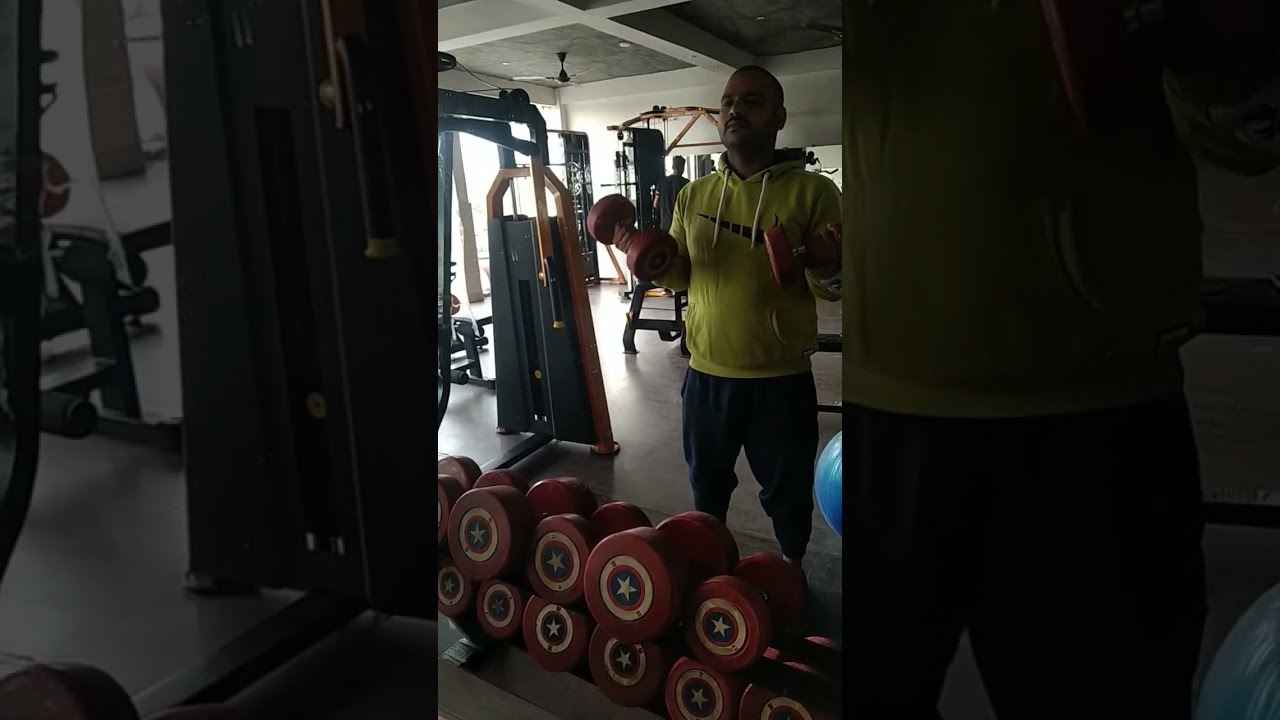This striking gym photo captures a brown-skinned man with close-cropped hair and a mustache, engrossed in his workout. Positioned at the center third of the image, he stands in front of a rack of red dumbbells, performing curls with a pair of red weights prominently adorned with the Captain America shield logo—red, white, and blue circles encircling a white star. He sports a vibrant yellow (sometimes described as lime green) Nike hoodie and blue track pants. The background reveals a typical gym setting with various machinery on a gray concrete floor beneath a white ceiling fitted with large recessed fluorescent lights. Additionally, a fan is visible on the seemingly dark ceiling. Behind the man, there's another gym-goer, clad in a blue t-shirt, possibly engaged with cable equipment. The encapsulating frame features dim, enlarged sections of the main image: on the right, a zoomed-in view of the man’s hoodie and pants; on the left, a piece of gym equipment. This composition hints at the scene's dynamic and energetic ambiance, typical of a well-equipped fitness facility.